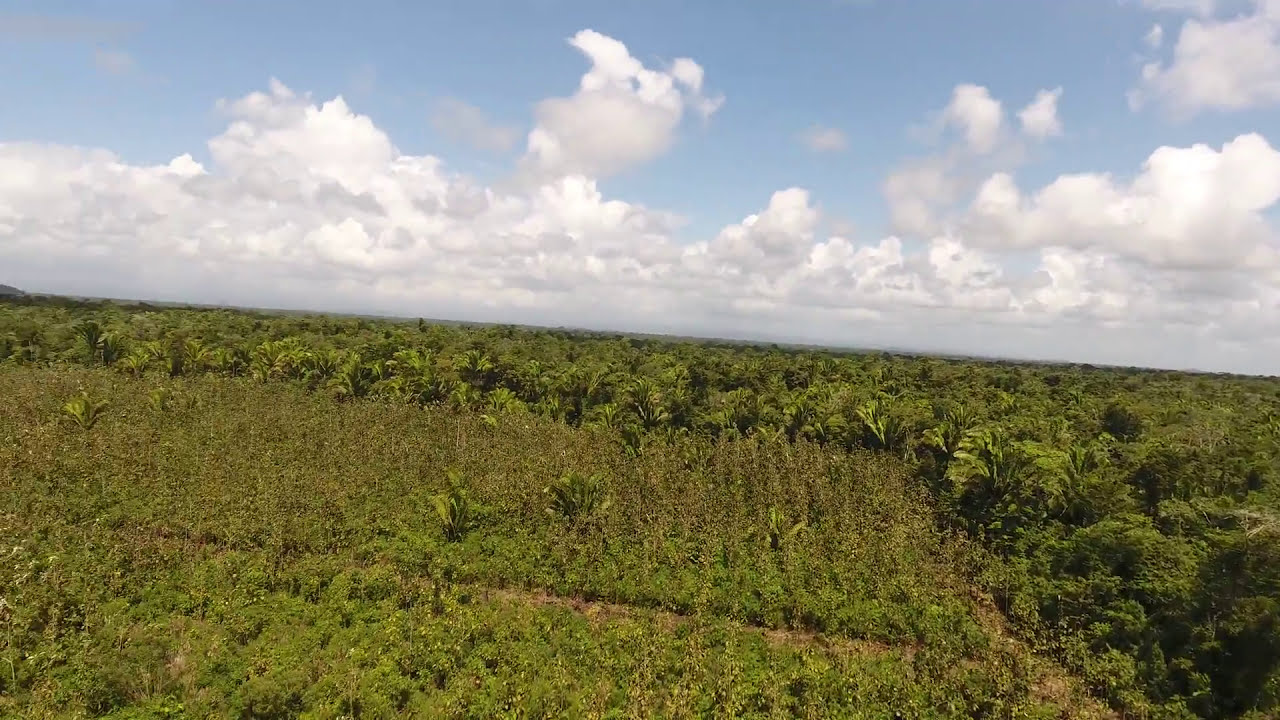The photograph captures a serene countryside setting dominated by natural landscapes. The sky at the top of the image is partly cloudy, filled with white, puffy clouds interspersed in a mostly blue expanse. The horizon line, located just above the middle of the image, marks the transition to a vast, grassy field that stretches as far as the eye can see. On the right-hand side, the field extends down to the bottom of the image, displaying lush green flora.

To the left, and occupying most of the frame but not extending to the extreme right, is a cultivated field that appears less dense and grassy. This field looks like it might have been planted in vertical rows, which have since become overgrown, making it difficult to identify the specific crops. The area around these plots is lined with large trees, suggesting a location that could be reminiscent of Southeast Asia, although no man-made structures or humans are visible. The overall scene is one of quiet natural beauty, with a garden area nearer the foreground, appearing slightly overrun with weeds, seamlessly blending into the verdant fields beyond.